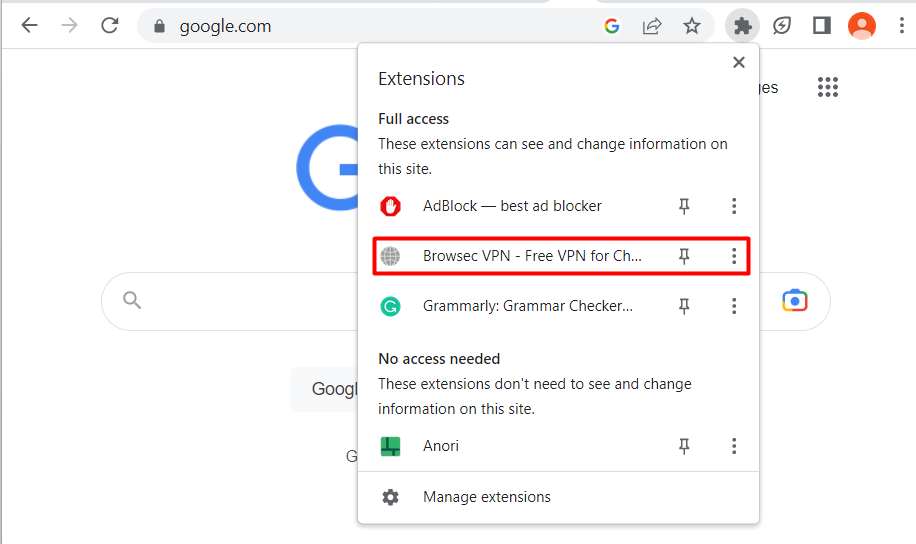This image features a web browser displaying a pop-up menu. At the top of the pop-up, the heading reads "Extensions." Below this heading, there are several entries listed. The first entry says "Full Access," followed by another entry labeled "Ad Block." Next, there is an entry for "Browser VPN," highlighted within a red rectangle. Below that is an entry for "Grammarly," described as a grammar checker. Following these, there is a section titled "No access needed," indicating that the listed extensions do not need to view or change information on the site. Under this section is an entry for "ANORI," and below that, an option labeled "Manage Extensions."

In the top-left corner of the browser, navigation icons are visible, including a back arrow, a forward arrow, and a refresh icon. To the right of these icons is the URL field, which displays "google.com." Further to the right, a series of small icons is present, including an orange profile picture icon.

The pop-up partially obscures the Google homepage. Only the uppercase blue "G" from the Google logo is visible on the left, and half of the search bar is still in view. The entire scene is set against a white background.